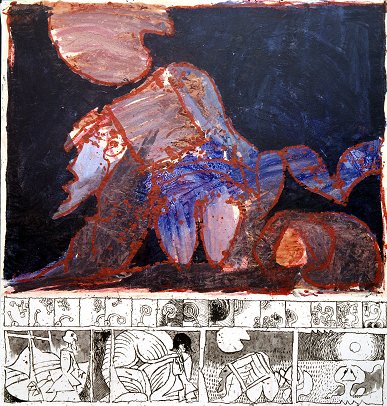The image depicts an abstract, seemingly ancient-style drawing on a dark, almost black background. The upper two-thirds of the artwork is in vibrant colors, featuring what appears to be a disjointed, anthropomorphic figure. The figure has a face on the left, a body suggesting movement, and limbs outlined in red and blue hues, reminiscent of primitive cave drawings. Stylized figures of a large and small animal, potentially with a moon in the sky, are outlined in orange crayon with blue and brown fills.

Below this colorful scene, a black-and-white comic strip-like section spans the width, comprising 16 small square frames filled with various abstract shapes and squiggly, flowery patterns. At the very bottom, there are four larger boxed panels. These panels feature a variety of unclear images, including a figure with what looks like a rack behind it, a large circular item possibly depicting a woman, an abstract fish, and another indeterminate shape that might resemble an abstract speech or symbol.

The overall piece gives an impression of movement and narrative, blending primitive art with a modern, comic-strip storytelling style.